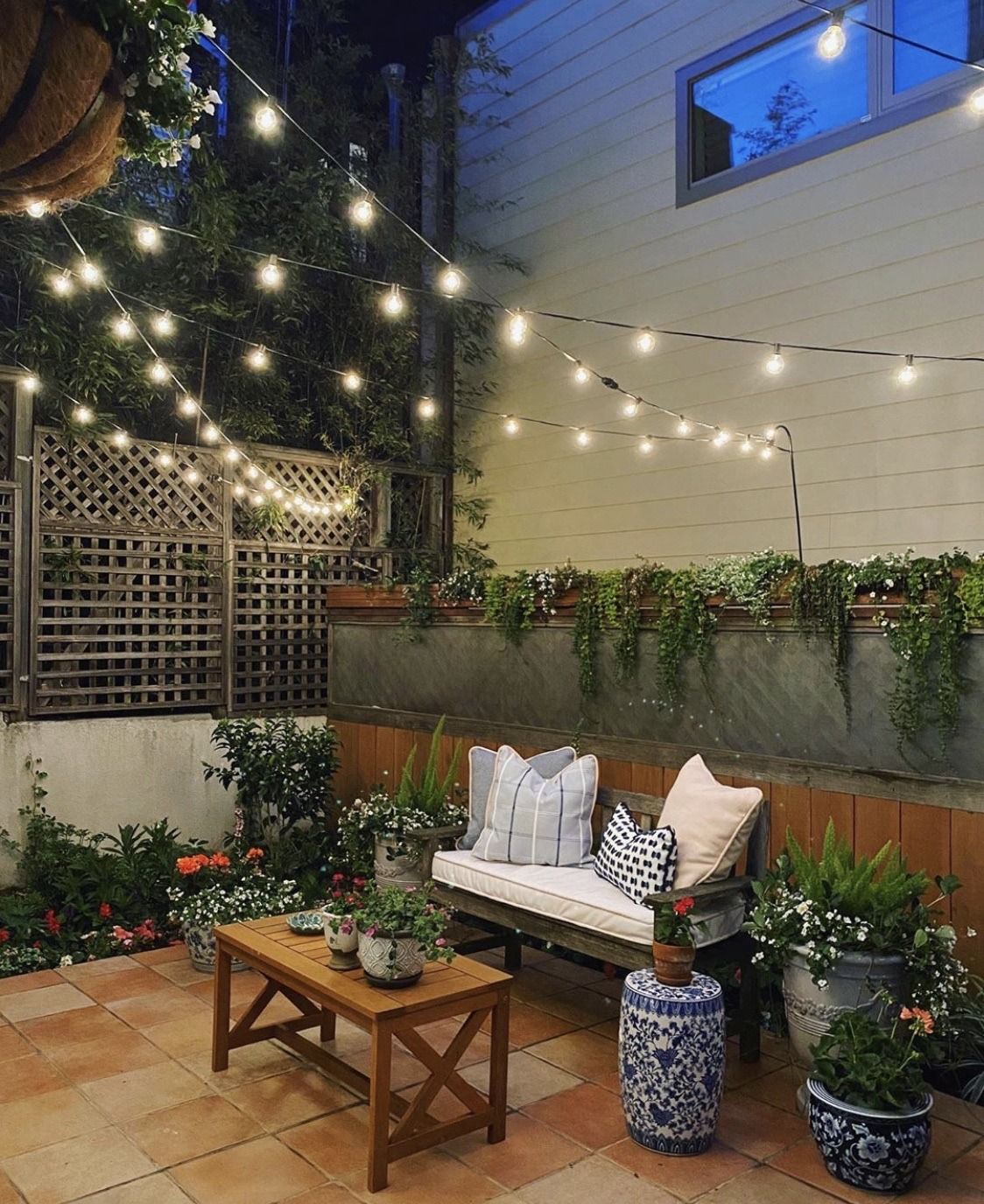The photograph captures a serene domestic courtyard or backyard patio, adorned with a variety of beautiful features that contribute to a peaceful, inviting scene. Dominating the center of the image is a wooden bench, roomy enough for two and accented with a comforting mattress and several throw pillows. The bench, made of dark, rustic wood, stands in contrast to the lighter, more modern wooden table positioned just in front of it. Together, the bench and table rest on a floor of terracotta tiles.

The courtyard is thoughtfully decorated with numerous potted plants, primarily housed in intricately detailed blue and white pots that add artistic flair. Both standing and hanging plants enhance the natural ambiance. Surrounding the seating area, lush greenery is visible, with plants not only confined to pots but also thriving in the ground and cascading from planters affixed to the walls.

Twinkling string lights, suspended on wires stretching across the courtyard, add a magical touch, illuminating the scene softly. Behind the bench, a combination of wooden fencing and a cement wall adds structure to the space, with flowering plants and vines spilling gracefully over the edge. A lattice fence at one end and a verdant flower bed filled with diverse blooms further enrich the charming, tranquil atmosphere.